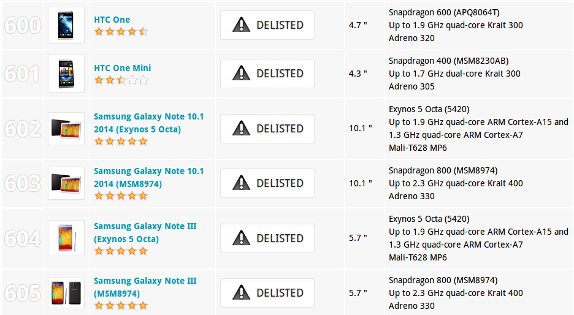The image depicts a detailed chart with six rows and five columns. The chart's background is grey with white cells, outlined in grey. The first column is titled "600," though it's faint. 

- **Row 1**:
  - **Column 1**: The number "600" in a faint, white text on a grey background.
  - **Column 2**: A small, unidentifiable icon within a square.
  - **Column 3**: The text "HTC1" accompanied by a rating of 4.5 stars.
  - **Column 4**: A black triangle with a white exclamation mark, followed by the term "delisted."
  - **Column 5**: Details of size and specifications: "4.7 inches" and "Snapdragon 6, APQ8064T, up to 1.9 GHz quad-core, KRLT3DD, Adreno 320".

- **Row 2**:
  - **Column 1**: The number "601".
  - **Column 2**: An image icon.
  - **Column 3**: The text "HCT1 mini" with a rating of 2.5 stars.

This pattern appears to repeat, with each row providing specific data points like device identification, ratings, status, and technical specifications.